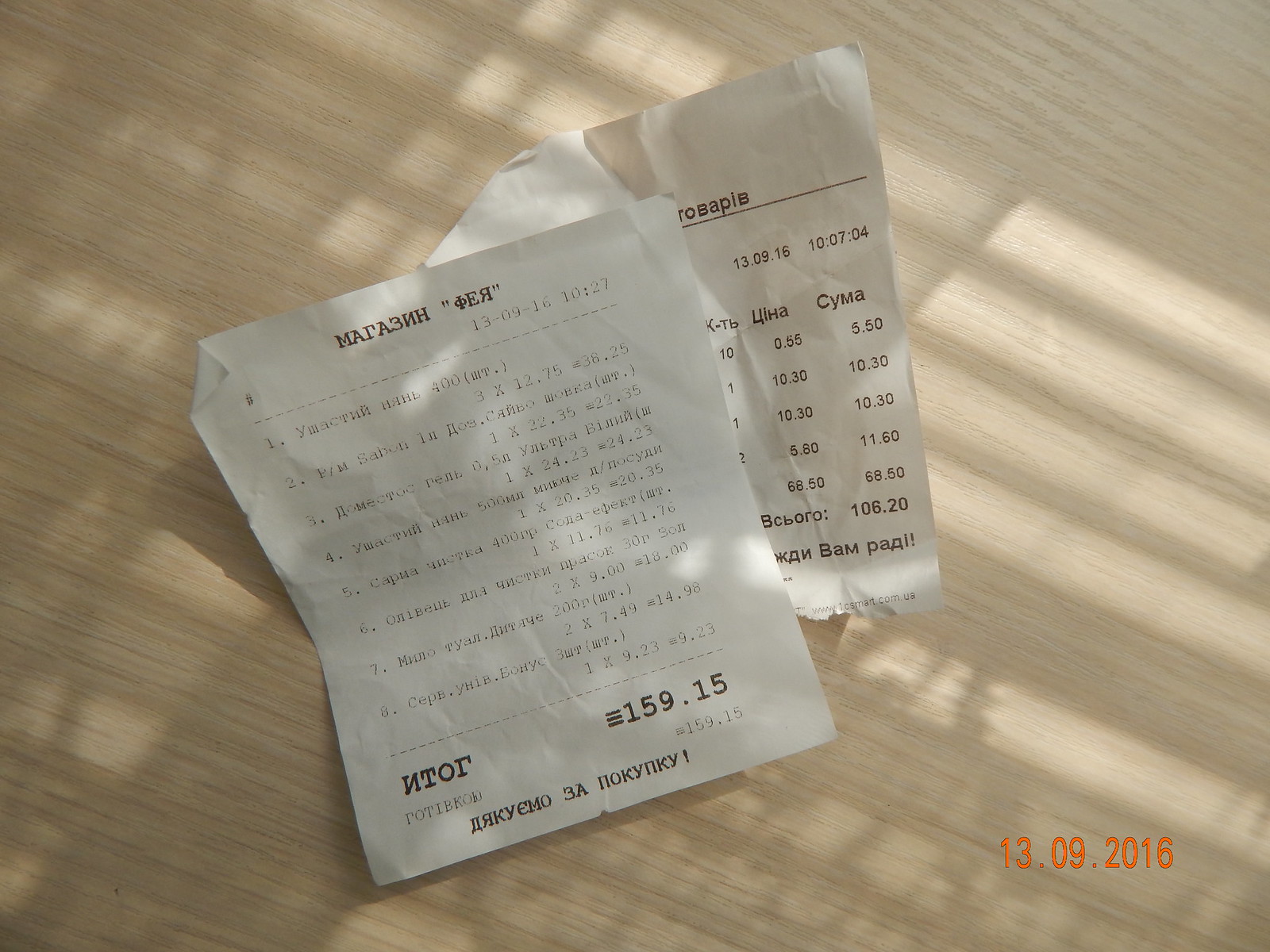This overhead photograph captures two paper receipts written in Russian, placed on a light beige, diagonally-patterned wooden surface, resembling a floor or table. The receipts, printed on white paper with black lettering, show line items with prices beneath them and a bolded total at the bottom. The leftmost receipt is stacked on top of the rightmost receipt, partially obscuring it. The top receipt lists eight items totaling $159.15, while the visible portion of the bottom receipt shows five items totaling $106.20. Light filters through vertical blinds, casting shadows across both the receipts and background. An orange digital timestamp in the bottom right corner of the photograph indicates the date as 13.09.2016.